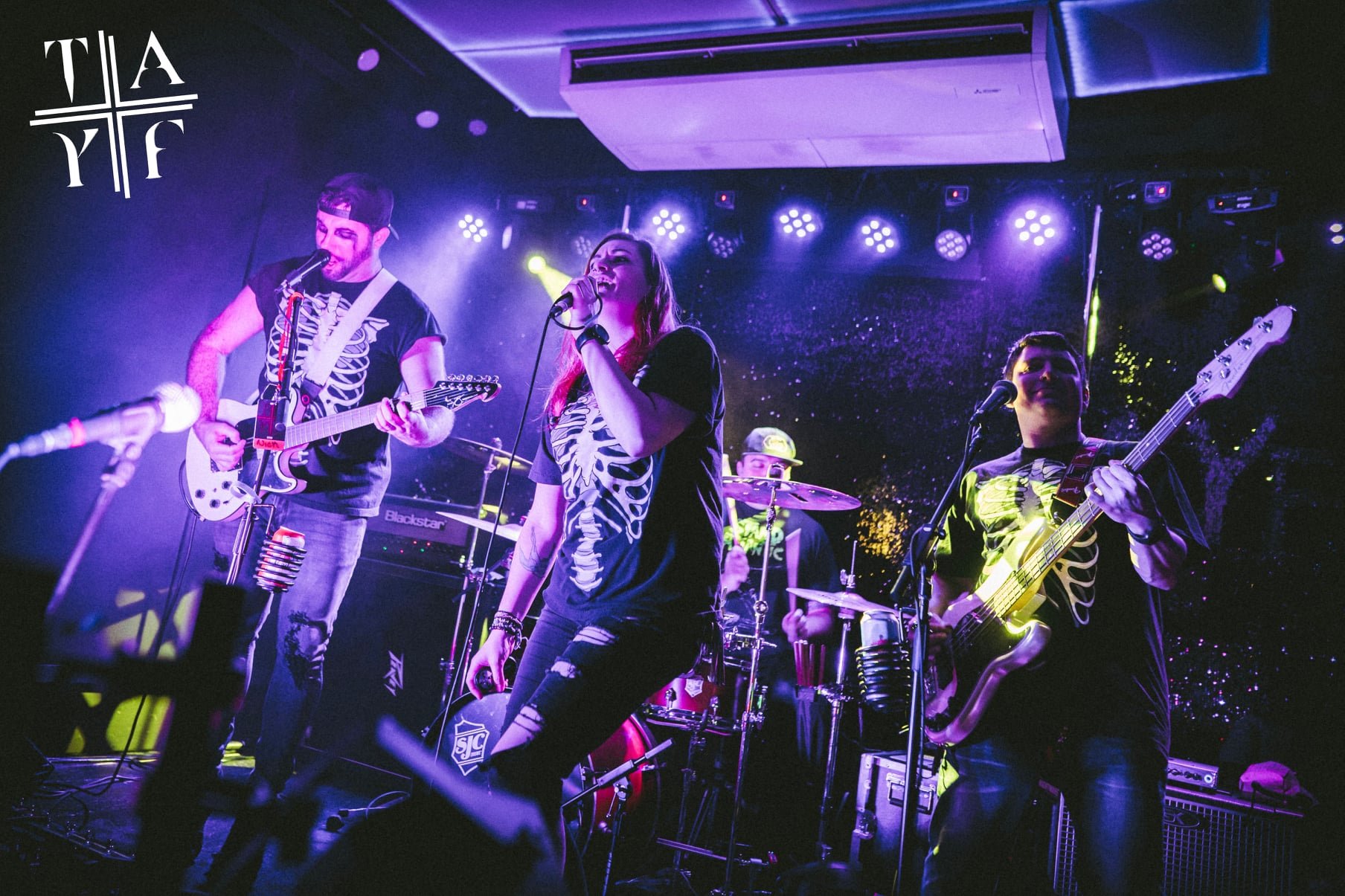The image captures a dynamic moment at a concert featuring a band of four members, all dressed in matching black t-shirts adorned with white skeleton designs and wearing ripped jeans. From left to right, the band members include a male bassist with a backwards hat who is providing backup vocals, a female singer with long red hair and bracelets passionately singing into the microphone, and a male guitarist who is shorter and appears to be deeply immersed in his music. Standing at the back, the drummer sports a black cap and a t-shirt with lime green lettering, and his red drum kit can be seen behind him. The band's logo, "T-A-Y-F," marked by a crosshatch separating each letter, is prominent in the corner of the stage. Blue and purple lighting create a vivid, colorful atmosphere, casting a tint over the performers and highlighting their movements on a relatively small stage. The dark background, possibly indicating a nighttime outdoor concert or a dimly lit venue, accentuates the vibrant hues, giving the entire scene a surreal, glowing effect.